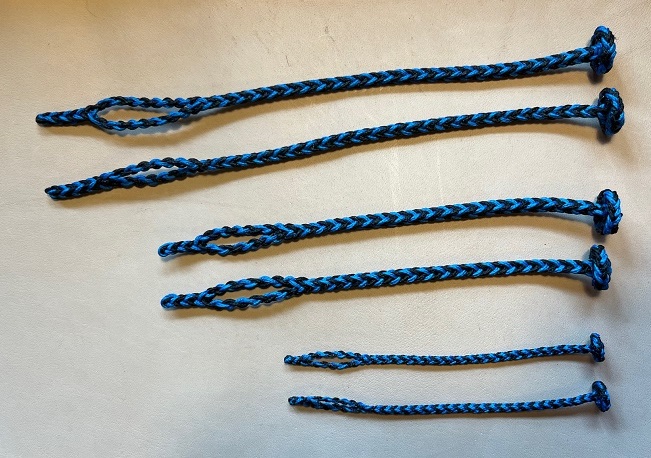The photograph showcases six blue and black braided rope fasteners, meticulously laid out on an off-white surface, possibly a table or floor. These fasteners are similar in function to bungee cords but do not stretch. They are organized into three pairs, each pair consisting of identical sizes: the smallest at the bottom, medium in the middle, and the largest at the top. The unique design features a loop at one end and a flattened "button" made of braided rope at the other, allowing them to form a secure closed system by threading the button through the loop. Ideal for various purposes such as securing items, hanging objects, and even sailing, these fasteners offer a versatile and sturdy solution.